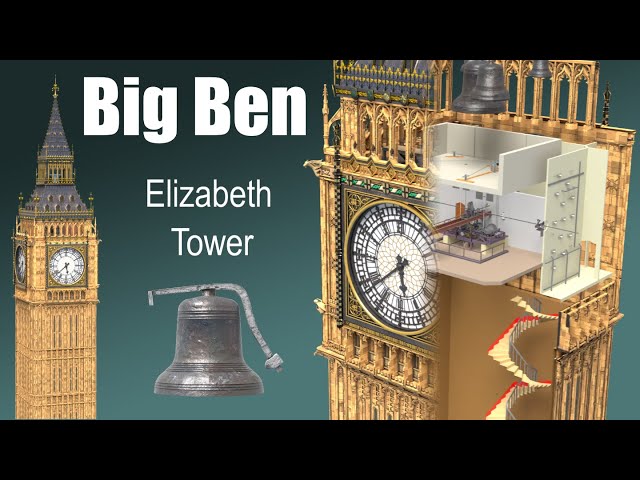The image depicts a computer-generated illustration of Big Ben, also known as Elizabeth Tower, in London. Dominating the left side of the image is a detailed view of the iconic clock tower, showcasing the top half with its prominent clock face set at 5:30 and its distinct steeple. The clock tower is depicted in yellow and accompanied by white lettering reading "Big Ben Elizabeth Tower," positioned above an illustration of the tower’s bell.

To the right, the image provides an insightful cutaway view of the tower's interior. This zoomed-in section exposes the inner workings of the structure, highlighting a cream-colored room that likely contains the mechanisms for operating both the bells and the clock. Within this cutaway, several bells are visible near the top, along with a long stairway leading downward. The cutaway is bordered by a black bar at the top and the bottom, adding a frame to this intricate cross-section of the tower, emphasizing the precision and complexity of its design.